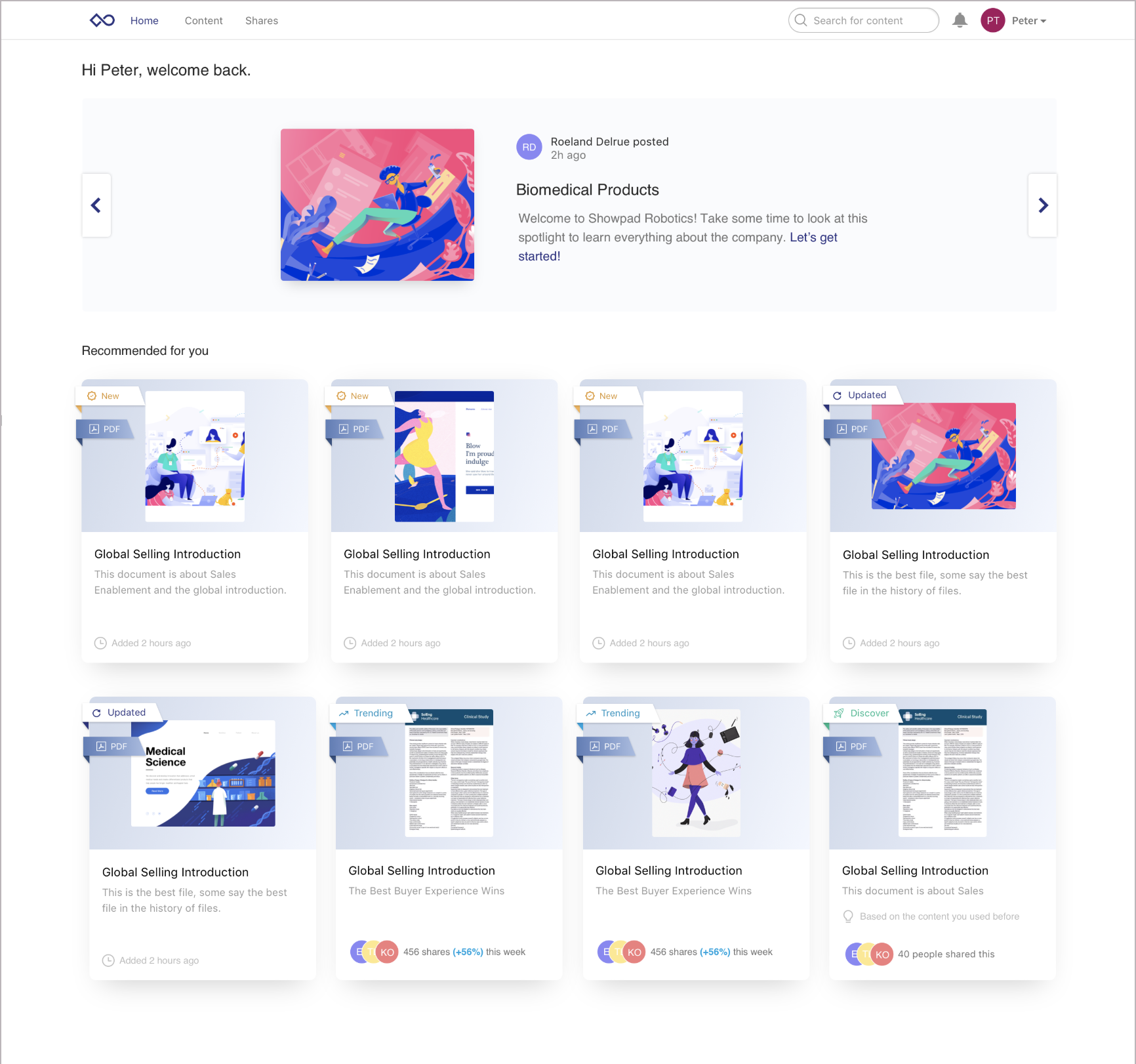This is a detailed screenshot from ShowPad Robotics. The main section of the image displays two horizontal rows of documents, with four documents in each row against a clean, white background. Each document is titled "Global Selling Introduction" and is accompanied by a colorful thumbnail drawing above its description.

In the upper-left corner of the page, a vibrant and abstract square illustration in pink, blue, and green catches the eye, though its exact subject is ambiguous. Just to the right of this image, text indicates that "Roland Del Rue posted two hours ago," followed by a message welcoming viewers to "Biomedical Products" and "ShowPad Robotics." The message encourages readers to explore the spotlight to learn everything about the company, ending with an inviting "Let's get started."

Additionally, in the top-left corner of the interface, a personalized greeting reads, "Hi Peter, welcome back," enhancing the user-friendly atmosphere. Welcome to ShowPad Robotics.